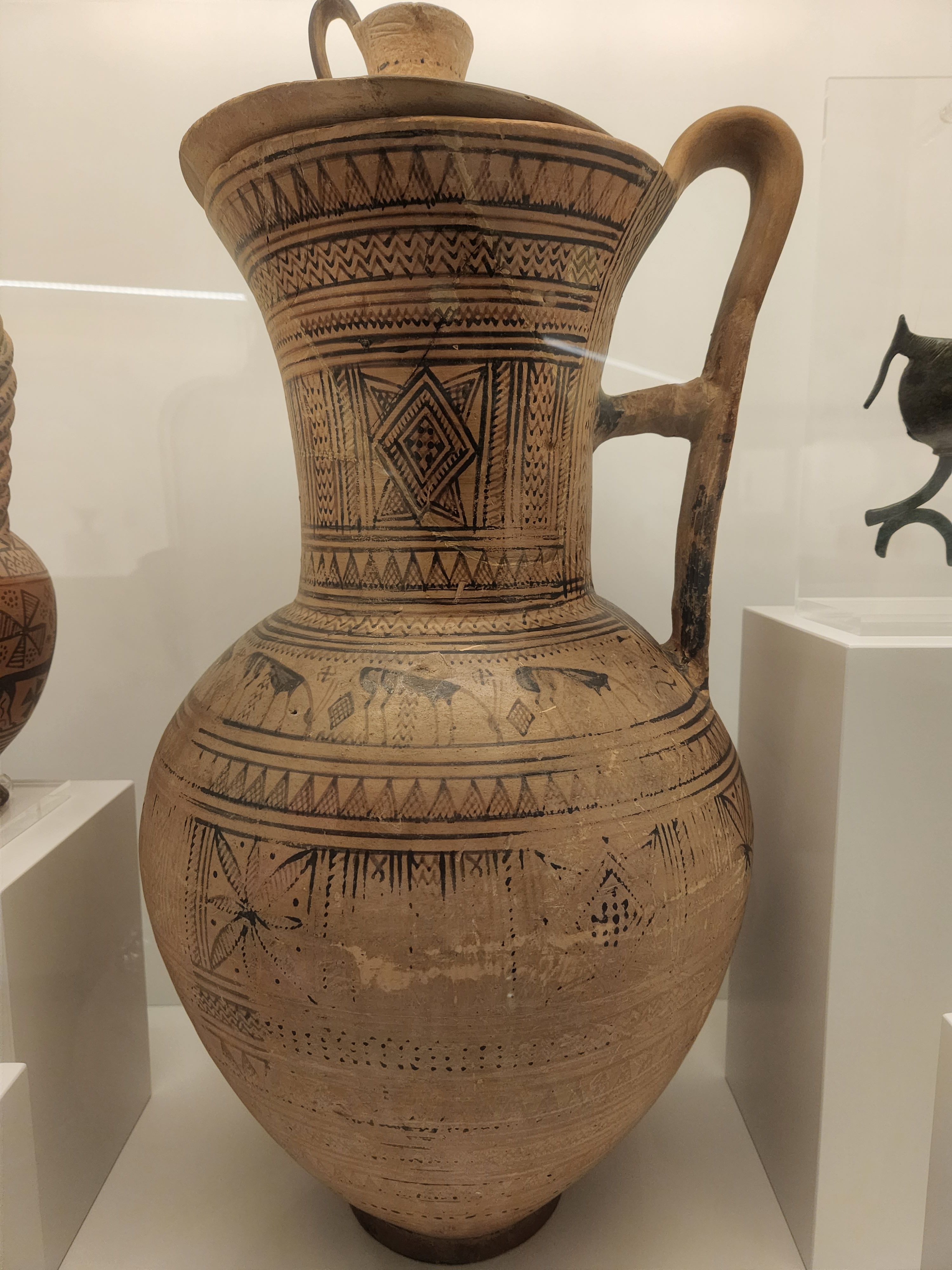In the image, we see a large, intriguing vase displayed in a glass cabinet within a museum setting. The vase has a distinct, rounded, teardrop shape at the bottom that gracefully transitions into a wide, bell-shaped upper section, culminating in a slightly flared rim. Crafted from ceramic or stone, the vase sports a light brown color and is adorned with black geometric and symbolic patterns.

The intricate black designs are predominantly concentrated on the upper portion of the vase and include a mix of zigzags, triangles, diamond shapes, wavy lines, and what appear to be hieroglyphic-style horses. The patterns are varied, with some resembling stacked triangles akin to candy corn, and others depicting chevron shapes and stacked lines. While the top part of the vase's design appears more detailed and intact, the bottom part shows signs of fading, indicative of the vase's age and historical significance.

Additionally, the vase features a prominent, looping handle on one side, starting from the belly of the vase and arching up before curving back down to meet the lower portion. The handle creates a bifurcated space, adding to the vessel's visual complexity. Another distinctive feature is the vase's lid, which is slightly off-center and has a handle that resembles a coffee cup's handle set on a plate, allowing for an easy grip.

The background of the display includes a white base and two square white pedestals on either side, emphasizing the vase's central position and highlighting its importance as an artifact. The overall setting, the craftsmanship, and the design motifs suggest a possible origin in the southwestern United States, with influences akin to Native American pottery, showcasing intricate geometric patterns and cultural depictions.